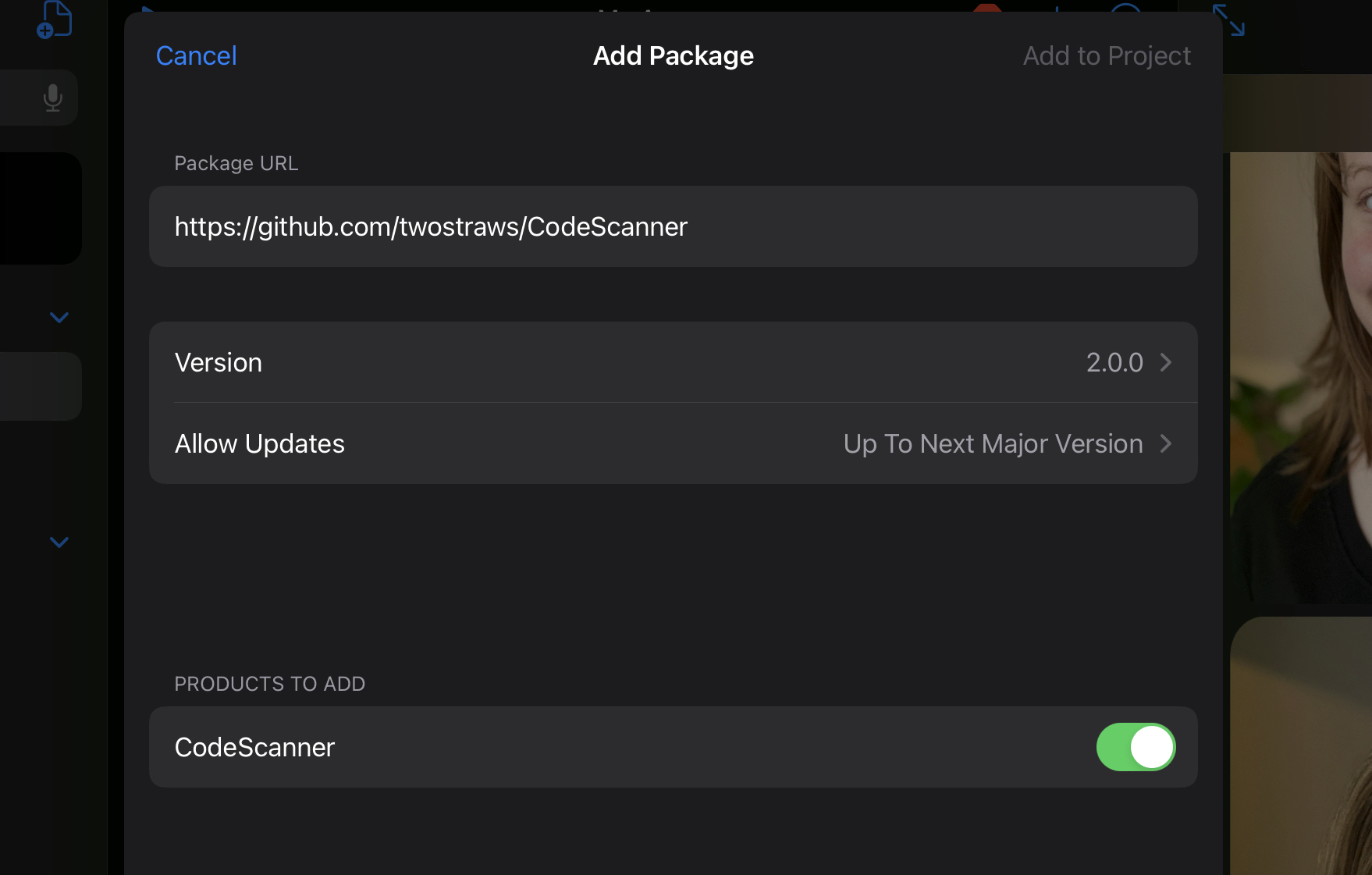A detailed descriptive caption for the screenshot could be:

---

The image depicts a user interface overlay on a webpage, obscuring most of the underlying content. The webpage itself features a predominantly gray color scheme with blue accents. On the right-hand side, partially visible thumbnails suggest media content, displaying part of a young girl with brown, shoulder-length hair, wearing a black shirt.

The overlay interface is centrally focused around configuring a package, titled "Add Package." At the top of the interface, navigation options include "Cancel" on the left and a faded "Add to Project" on the right. 

The main section of the overlay provides detailed configuration fields:
- "Package URL" with an inserted GitHub link.
- "Version," specified as 2.0.0.
- "Allow Updates" set to "Up to next major version."

Further down, there is a section labeled "Products to Add," with an entry named "Code Skin." A toggle button next to this entry is activated, indicated by its green color and position turned to the right.

---

This caption offers a thorough description of the screenshot, detailing both the visible webpage elements and the content of the overlaying interface.